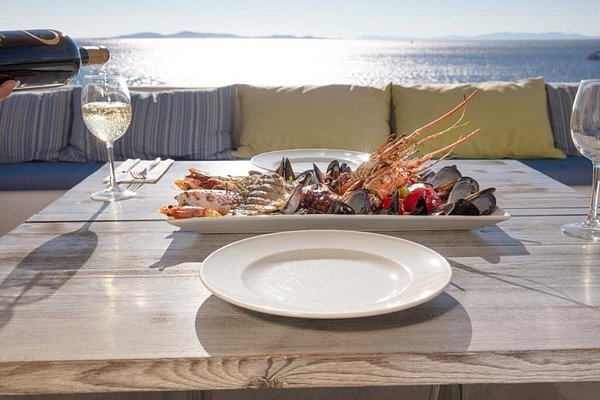This photograph captures an elegant outdoor dining scene set against the stunning backdrop of a large lake or sea. The scene is bathed in afternoon sunlight under a clear blue sky, with calm blue waters and distant mountains or landmasses visible across the shore. The dining setup features a light brown wooden table, which showcases a rectangular platter brimming with an assortment of seafood, including lobster, prawns, crab, clams, mussels, and possibly fish.

Two white circular plates are positioned on either side of the seafood platter. There are also two wine glasses on the table; one is empty while the other is being filled with white wine from a dark bottle held by a barely visible Caucasian hand. Complementing the lavish spread is the seating arrangement featuring a black bench-like sofa adorned with a mix of yellow and blue pillows, some of which display white and gray stripes.

The serene water, the sunlight reflecting off its surface, and the well-appointed table laden with delicacies all combine to create an idyllic and luxurious waterfront dining experience.